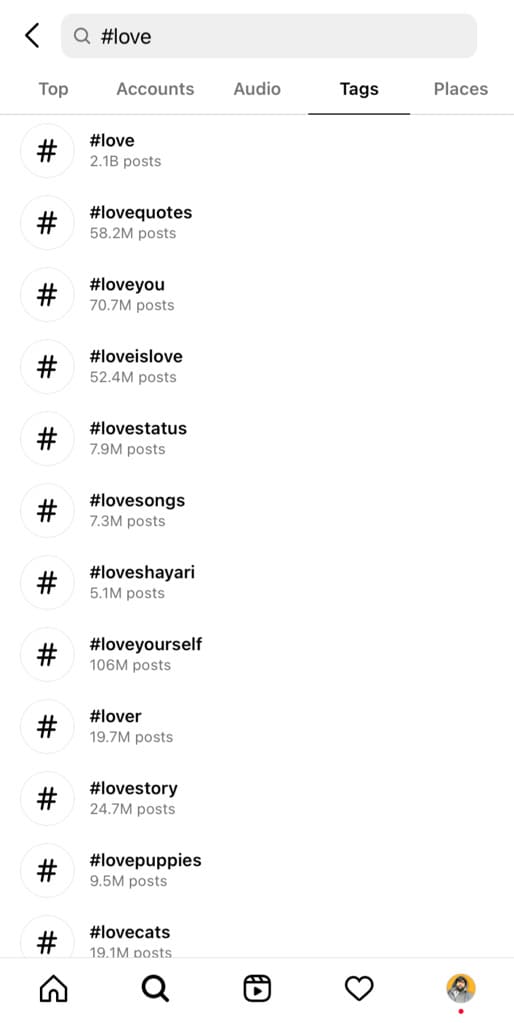A detailed screenshot from a smartphone's Instagram app interface is displayed. The image is vertically oriented, indicating it was captured from a mobile device. At the top of the screen, a prominent, long gray search bar is visible with the text "#love" entered. An arrow icon points to the left within this search bar.

Below, a set of search categories is presented in a horizontal menu: "Top," "Accounts," "Audio," "Tags," which is highlighted in bold and underlined, and "Places." This highlights that the current view focuses on the "Tags" option.

The middle section of the screen showcases a list of hashtags related to the search query '#love.' Each entry features an icon of the pound symbol on the left, followed by the hashtag's name and the number of associated posts on the right. The listed hashtags include:
- #love
- #lovequotes
- #loveyou
- #loveislove
- #lovestatus
- #lovesongs
- #loveshayari
- #loveyourself
- #lover
- #lovestory
- #lovepuppies
- #lovecats

At the bottom of the screen, the standard Instagram navigation bar is visible, showcasing five icons: a house for the homepage on the left, a magnifying glass for search, a square with a play symbol for Instagram Reels in the center, a heart symbol for liked posts, and finally, a circular profile picture representing the user's account on the right.